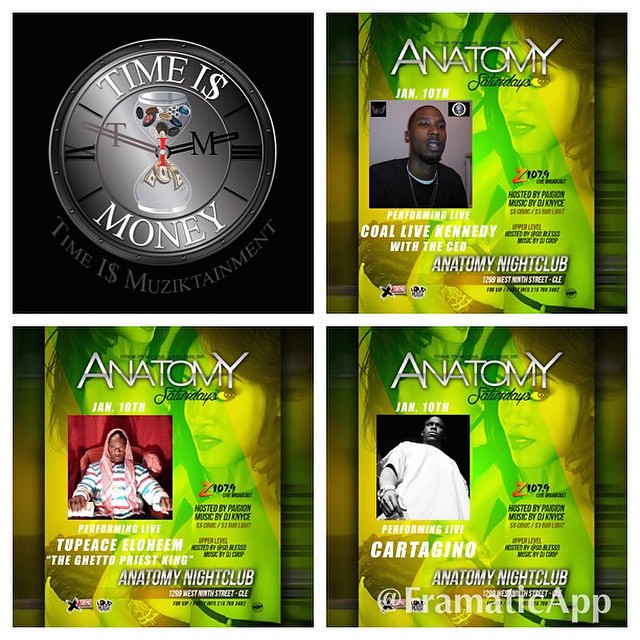This vibrant quartet of promotional flyers for Atonomy Nightclub, located at 1299 West 9th Street, provides an engaging preview of their upcoming event on January 10th. Each flyer reveals unique details about the performers and the nightclub's weekly event, Atonomy Saturdays. The upper left flyer features an artistic representation of an hourglass within a clock, emblazoned with the phrase "Time is Money." The upper right flyer, with its striking green background, announces the headline performer: Coal Live Kennedy, the CEO of Atonomy Nightclub, emphasized in bold green, yellow, and white lettering. The lower two flyers continue the theme, spotlighting different performers: Two Piece Ilomi, affectionately known as the Ghetto Priest King, and Cardigan L. Additionally, there's a subtle image of a woman in the background of these flyers, possibly indicating her involvement as a performer this Saturday. These posters collectively underscore the excitement of Atonomy Saturdays, now further enlivened by a sponsorship from Z107.9.